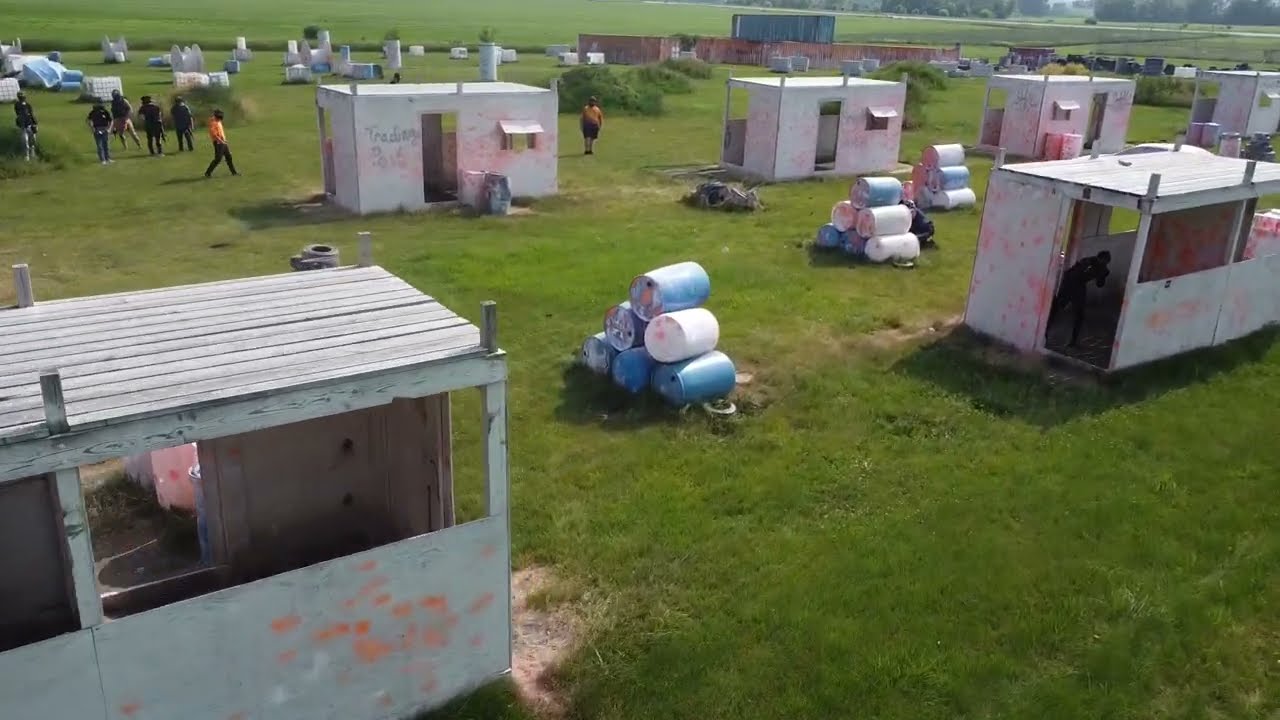The image depicts a large, sunny field of green grass interspersed with several makeshift shelters. These shelters, spaced about 15 feet apart and arranged in two rows, have open doorways and windows, but lack doors and glass. They appear to be basic structures made of wood, possibly providing minimal shelter from the elements. In the foreground, barrels painted blue and white are stacked in a pyramid shape between the shelters. Towards the middle left of the image, about half a dozen people, mostly in dark clothing with a couple in yellow hoodies, are standing and wandering around. The grass shows signs of dryness in some patches, particularly near the entrances of the shelters. In the far background, there are additional indistinct structures that suggest an industrial setting, with what might be metal, possibly railroad cars, further enhancing the scene's utilitarian atmosphere. Additionally, a few green bushes can be seen scattered throughout the area. The skyline is lined with distant trees, adding an element of depth to the photograph.